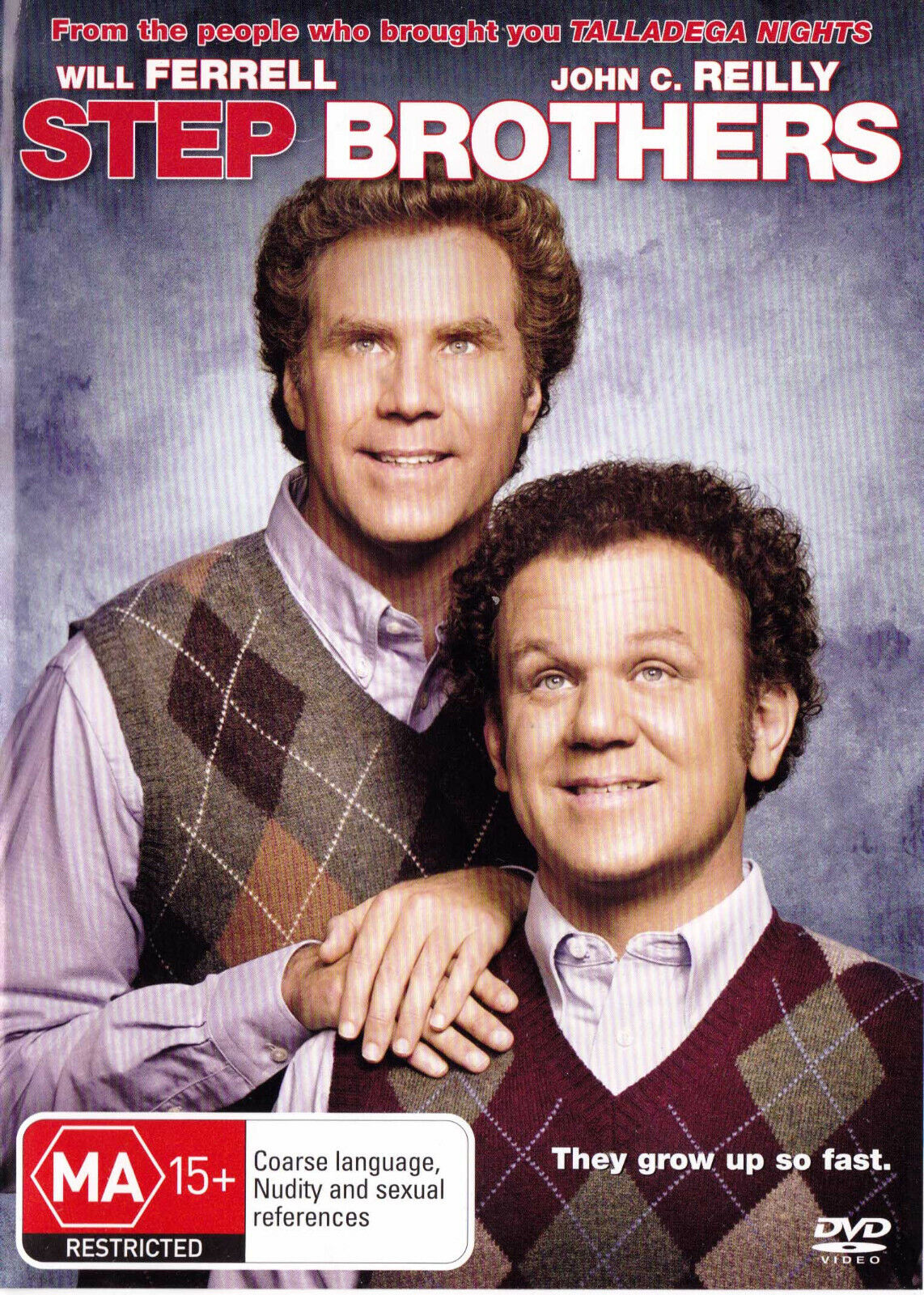The cover of the DVD for the movie "Step Brothers" features the two main actors, Will Ferrell and John C. Reilly, in a memorable pose. Will Ferrell is standing behind John C. Reilly, with his hands gently placed on John C. Reilly's right shoulder. Both actors are clad in Argyle V-neck sleeveless sweaters over collared, button-down, long-sleeved shirts. Will Ferrell is positioned on the left, while John C. Reilly is on the right. The top of the cover prominently displays "Step Brothers" in all capital letters, with "Step" in red print and "Brothers" in white print. Above the title, in smaller red letters, it reads, "From the people who brought you Talladega Nights." The names of the actors are printed above this, with Will Ferrell on the left and John C. Reilly on the right. The bottom left of the cover includes a parental advisory sticker marked "MA 15+ Restricted," indicating coarse language, nudity, and sexual references. The bottom right corner features the tagline, "They grow up so fast," in white letters, and a small "DVD Video" logo is present in the lower right part of the image.